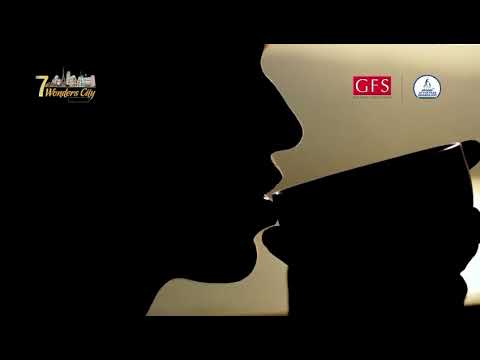The image is a horizontally aligned rectangle featuring the side view outline of a person's face, fully blacked out with details only visible in silhouette. The individual, likely a male, has their mouth slightly open and is holding a coffee mug near their lips. Only the shape of the face, hand, and cup are visible. The background of the image is a grayish beige. In the upper left corner, there is a gold logo with the words "Seven Wonders City" and a small cityscape illustration. In the top right corner, there is a red rectangle containing the white capital letters "GFS." Adjacent to this is a circular logo on a white background with an indistinguishable image and text. Thick black horizontal borders frame the top and bottom of the image.